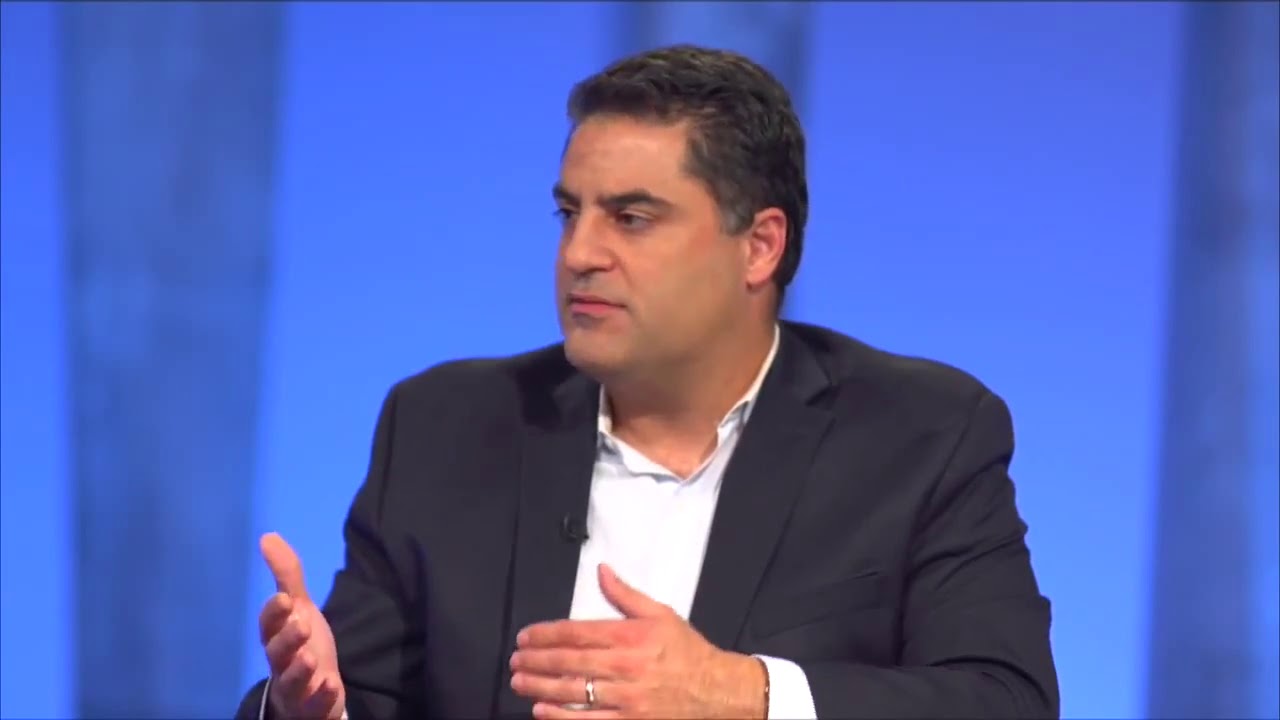This detailed indoor photograph captures Cenk Uygur, a newscaster from The Young Turks YouTube news network, seated centrally in the frame. He is dressed in a black suit blazer and a white collared shirt, notably without a tie, and a small microphone is affixed to his coat. His facial features are clearly visible; he has a peach complexion and black hair, and his mouth is closed as he appears to be in the middle of a conversation, looking towards his right. His hands are positioned in front of his body, gesturing slightly, with a ring adorning one of his fingers. The backdrop consists of a blue gradient with darker shaded lines, which is blurred out, drawing attention to Cenk as he seemingly prepares to speak. The image focuses entirely on him, emphasizing his poised demeanor amidst what appears to be a newscast or debate scenario.